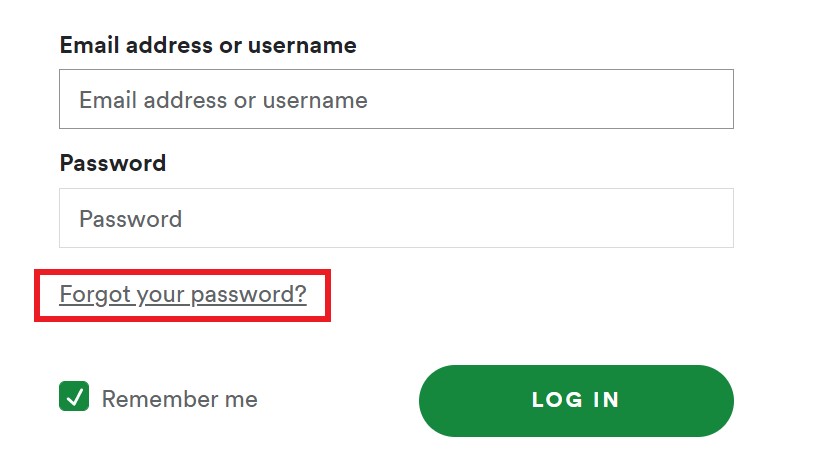The image displays a login form set in landscape mode. The background of the form is entirely white. At the top, the first row features a bold, dark black label that reads "Email Address or Username." Directly beneath this prompt is a light gray input field where users can type in their email address or username; the placeholder text in the box also says "Email Address or Username" in gray.

The following section has another dark black bold label, which reads "Password." Below this is another light gray input box marked with the placeholder text "Password," indicating where users should type their password.

Highlighted in a red rectangle below the password field is the underlined text "Forgot your password?," indicating a clickable link to assist users who need to recover or reset their password, despite the absence of the typical blue hyperlink color.

Further down, on the lower left, there is a green checkbox, labeled "Remember me," which has been checked off.

On the bottom right side of the form, a prominent green button with white text states "Log in."

In summary, this login form prompts the user to enter their email or username and password, offers an option to remember their credentials, and provides a reset password link. The "Forgot your password?" feature stands out in red to ensure users can easily identify the essential password recovery function.